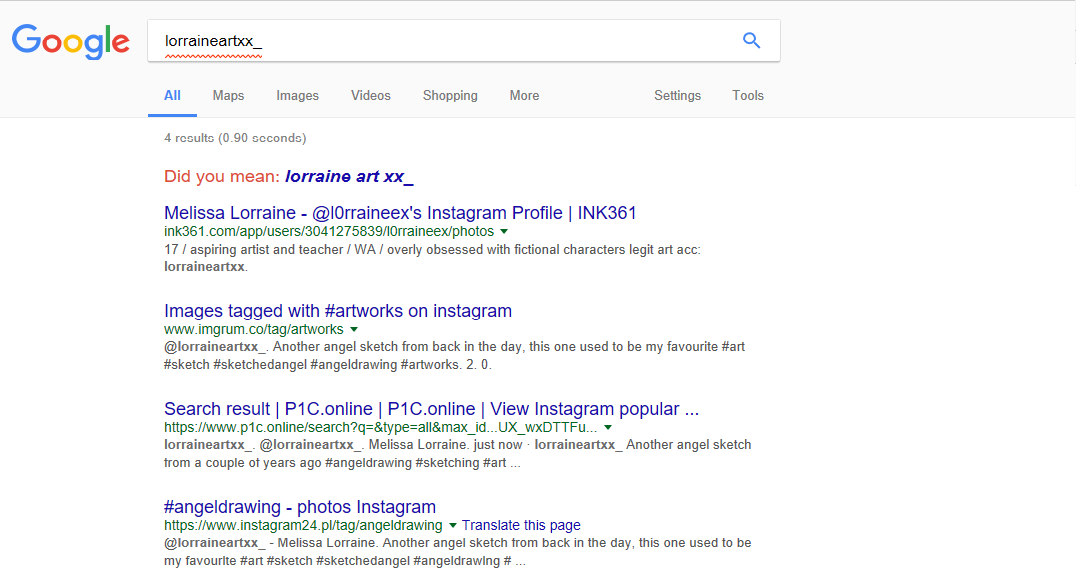The image depicts an older screenshot of a Google browser interface, characterized by the classic Google logo in the upper left corner. The logo features a blue capital "G," followed by "oogle" in red, yellow, blue, green, and red respectively. 

To the right of the logo is the search box containing the query "LorraineArtXX_" (spelled as L-O-R-R-A-I-N-E-A-R-T-X-X underscore). This query is underlined with a red squiggly line, indicating a possible misspelling. 

Above the search results are various tabs labeled "All," "Maps," "Images," "Videos," "Shopping," "More," "Settings," and "Tools," with the "All" tab currently selected. The search results header notes "For Results (.9 seconds)." 

Below this header, Google suggests, "Did you mean LorraineArtXX_?" 

The search results include a range of links with snippets of blue text. Some of the notable links are:

- "Melissa Lorraine, at LorraineX's Instagram profile, Inc. 361"
- "Images tagged with hashtag artworks on Instagram"
- "Search result, p1c.online, view Instagram popular"

These results appear to be related to social media profiles and tagged artworks, hinting that "LorraineArtXX_" is likely associated with artistic content or a social media handle.